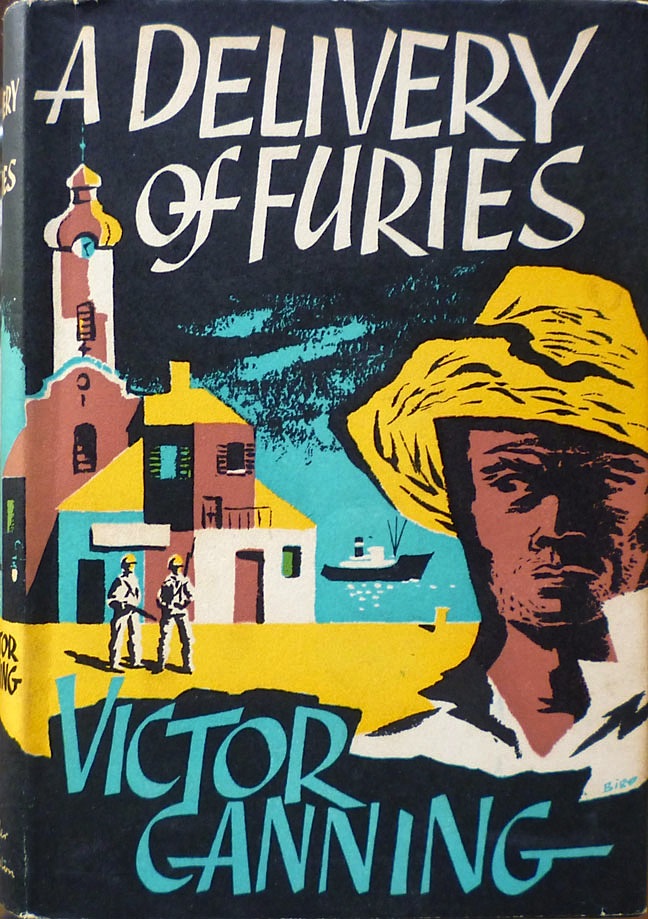This is the cover of a book titled **"A Delivery of Furies"** by **Victor Ganning**, prominently displayed in bold white capital letters at the top against a stark black background. Below the title, the author’s name is written in turquoise against the same dark backdrop. 

The central image is complex and evocative, featuring a multi-colored building that resembles a church with a steeple topped by a cross. The building, situated on the left side of the cover, is intricately detailed with a combination of pink, yellow, and blue hues, as well as a clock in the middle of the steeple. 

In the scene’s background, there's a turquoise blue body of water, through which a black and white ship or steamboat is sailing. In front of the building, stand two men dressed in white clothing and yellow hats, seemingly armed with rifles, suggesting they might be military guards or soldiers. 

Dominating the foreground to the right is a larger image of a black man wearing a large yellow sun hat. His face is shaded, adding an element of mystery and concern as he gazes sideways, partially towards the church and the men in front of it. The cover's styling hints at its old-fashioned, almost vintage aesthetic, reminiscent of classic hardcovers with paper dust jackets.